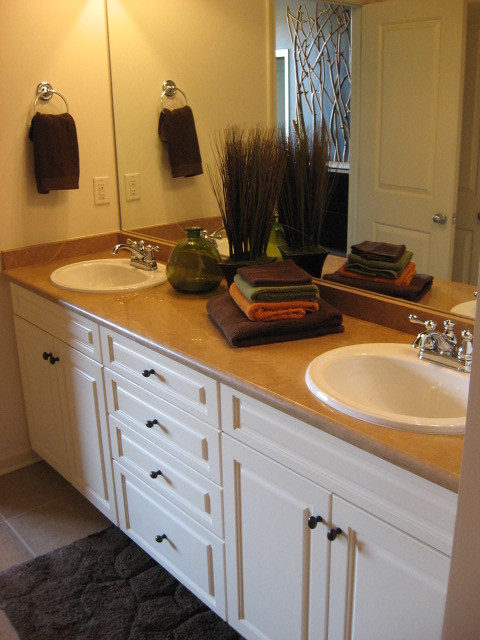A well-organized bathroom features a double vanity with white cabinets and brown countertops. The vanity has two evenly spaced, traditional white sinks with silver chrome faucets. In the center of the counter, between the sinks, neatly folded towels are stacked. At the bottom of the stack is a large brown towel, followed by an orange one, then a blue towel, and topped with another brown towel. Decorative touches include a vase holding an arrangement of twigs and another clear green vase, which stands empty, adding a subtle touch of color to the space.